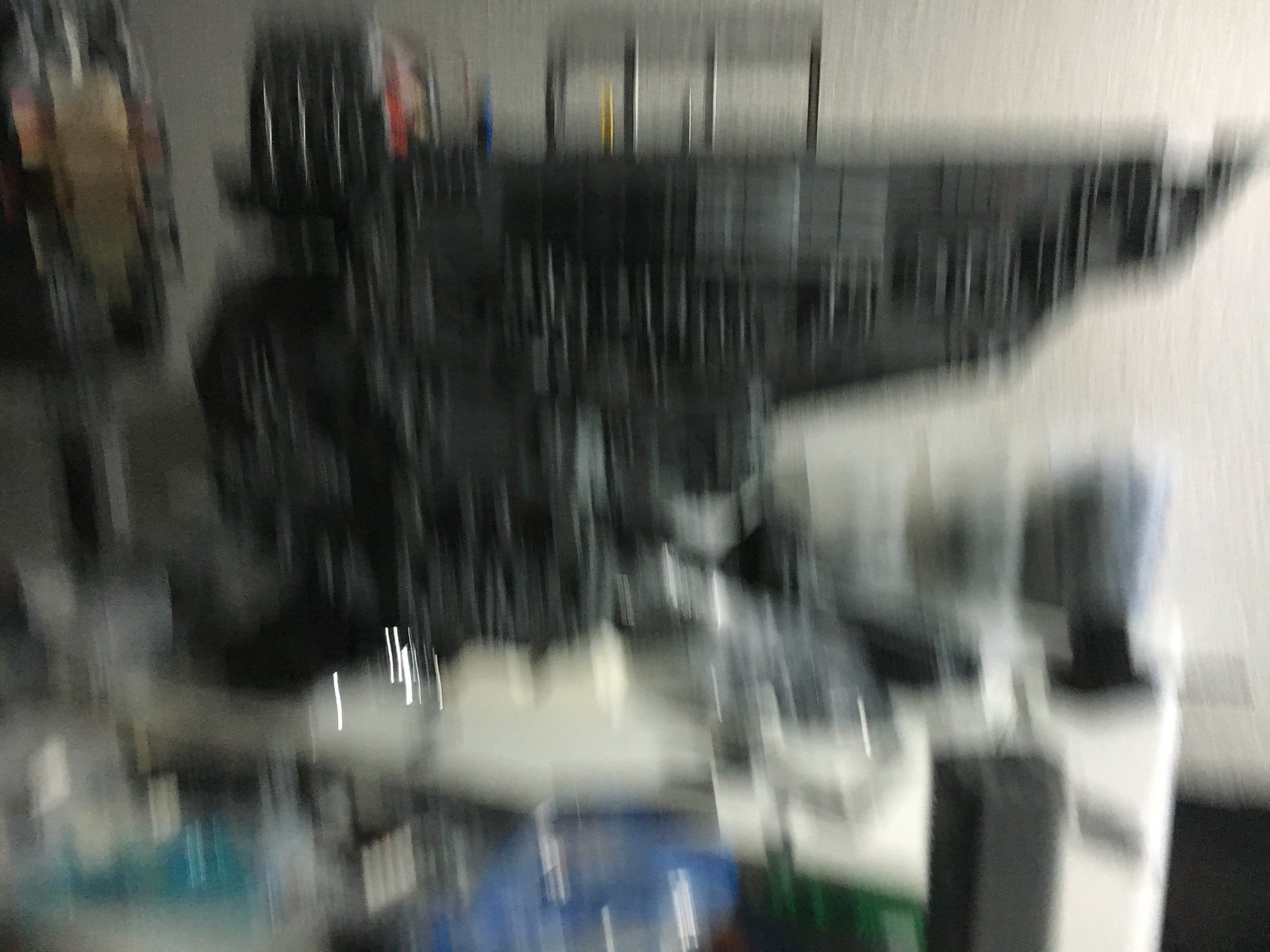This photograph, although very blurry and distorted, primarily features a large black object resembling a battleship, possibly constructed from Legos. The camera seems to have been shaken when the image was captured, contributing to the lack of clarity. Atop the battleship-like structure, there are noticeable accents in red, as well as slender objects in blue, yellow, and silver. The backdrop consists of a plain white wall, and the battleship appears to be situated on a white table. Surrounding it, various objects can be seen including some in black and white. Near the bottom of the image, there are shades of teal, blue, and green, adding a bit more color to the scene.